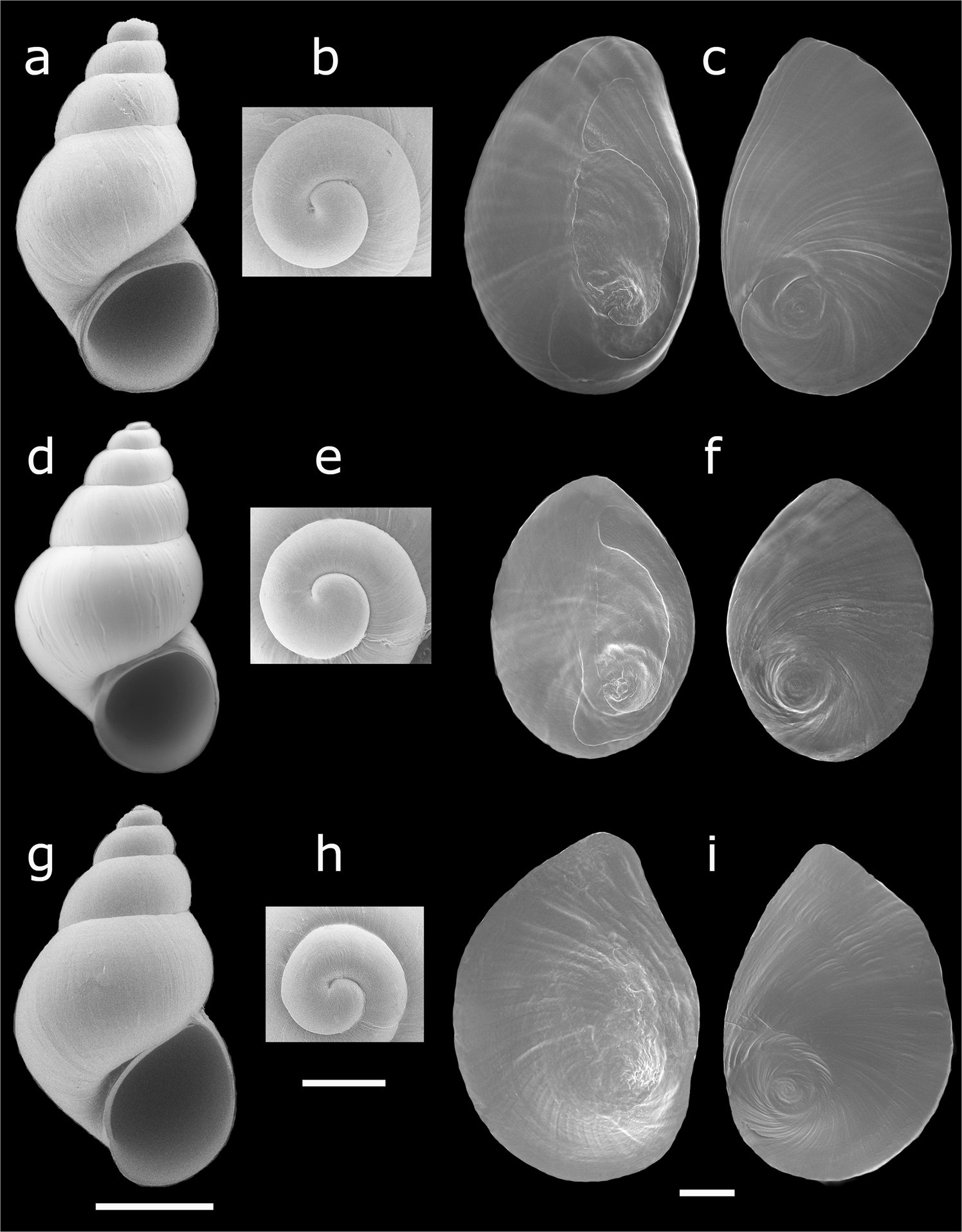This image is an intricately detailed poster featuring x-ray images of various seashells. Set against a black background, the poster presents three distinct columns, each illustrating different views of the shells. On the left side, under labels A, D, and G, are long views of small snail shells showing their openings. The middle column, labeled B, E, and H, displays top views of these shells, capturing the start of their spirals in tiny square x-rays. The rightmost column, labeled C, F, and I, features cross-sectional views that reveal an iridescent, see-through quality with an ivory color. Each image is captioned with letters ranging from A to I, providing a thorough and systematic visual study of the seashells. Additionally, horizontal white lines are placed beneath some of the images for emphasis.